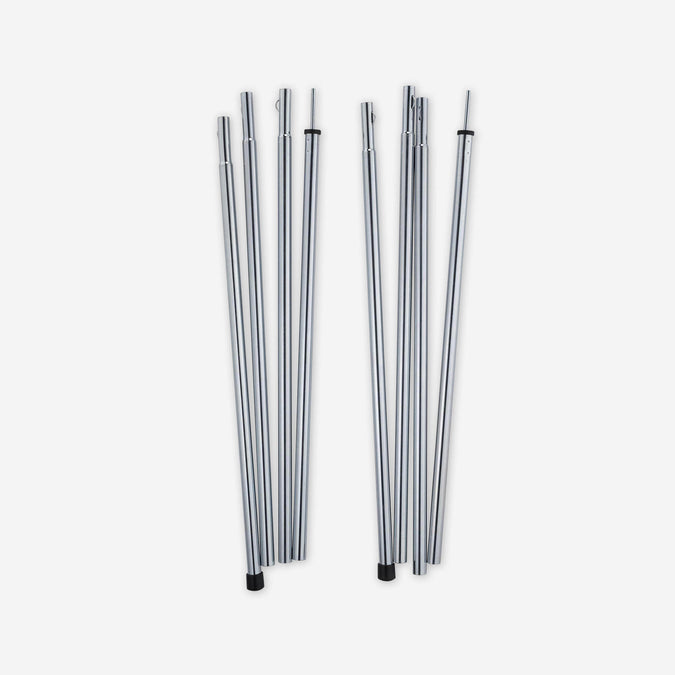The photograph features eight or nine silver-colored metal rods laid out on a white surface. The rods are organized into two groups, each array containing four segments. All rods have a collapsible feature where they can connect together, possibly utilizing a single tight elastic string, although this detail isn't visible. The bottom of several rods is finished with black rubber caps, while the other ends have open tips that could be narrower for connection purposes. Additionally, there are two rods with pointy ends. Small buttons on the rods pop out for secure assembly, allowing the segments to be easily taken apart and reassembled. They appear to be designed for easy transport and adjustable length, though their exact purpose is unknown.